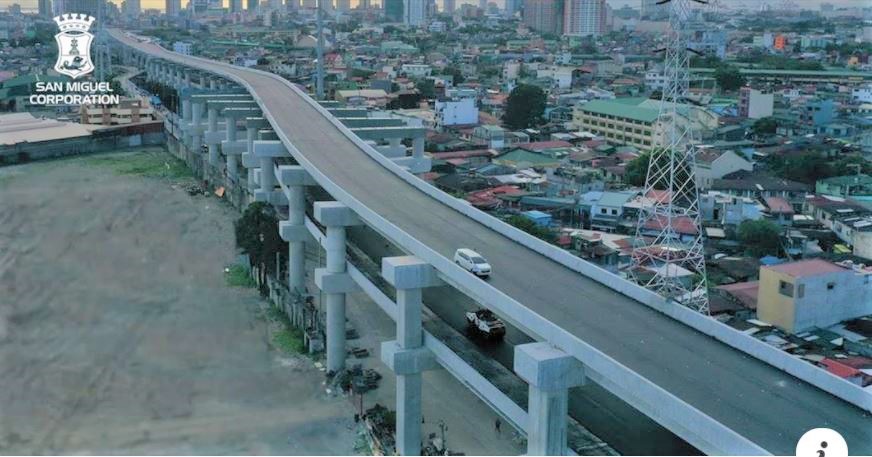An aerial photograph showcases a bustling metropolitan area dominated by a double-decker bridge with a black asphalt surface. This bridge spans diagonally from the bottom right to the upper left of the image, supported by large rectangular columns and dotted with vehicles, including a white minivan heading to the right on the top level and a black sedan on the bottom level. To the right of the bridge lies a sprawling cityscape with a mix of low-rise residential buildings, a motel, and a three-story structure resembling a parking garage with a light green roof. A prominent transmission tower stands tall in the bottom right corner. In the background, an array of towering skyscrapers forms the city's horizon. On the left side of the image, there's a vast, open, vacant lot providing contrast to the densely packed right side. The image features a palette of colors including brown, white, red, green, blue, and black. In the upper left corner, a white logo with a crown and a shield reads "San Miguel Corporation."